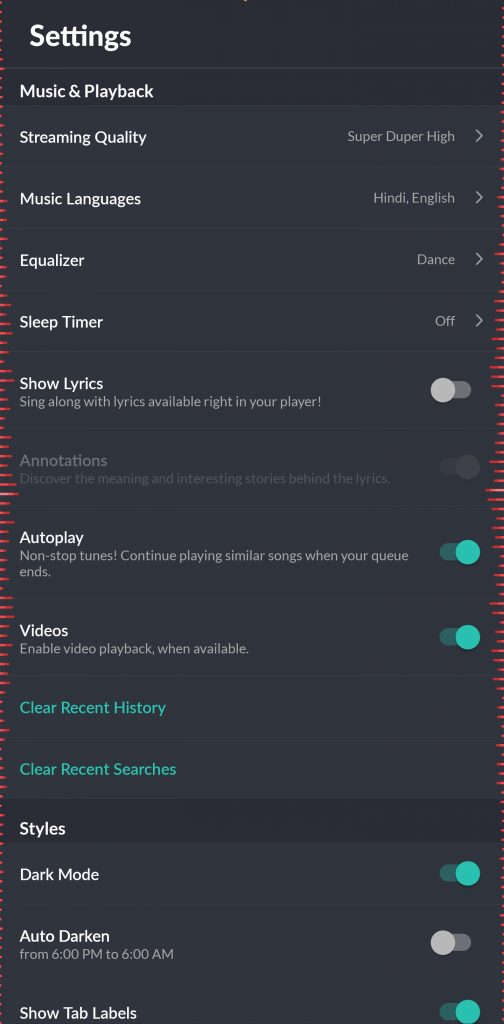This is an image of a settings page with a predominantly dark, grayish-black background and white font. There are multiple toggle switches, specifically seven, which can be toggled on and off. The settings page is divided into two main sections: "Music and Playback" at the top and another section below it.

In the "Music and Playback" section, the following options are presented:
- **Streaming Quality**: Set to "Super Duper High".
- **Music Languages**: Set to Hindi and English.
- **Equalizer**: Set to "Dance".
- **Sleep Timer**: Set to "Off".
- **Show Lyrics**: A description beneath this reads "Sing along with lyrics available right in your player", but this option is toggled off.

Below these, there are options for:
- **Annotations**: This option is grayed out and appears inactive.
- **Autoplay**: This option is toggled on.
- **Videos**: This option is toggled on.
- **Clear Recent History**
- **Clear Recent Search Option**

This detailed layout provides a comprehensive view of the settings available in the image.